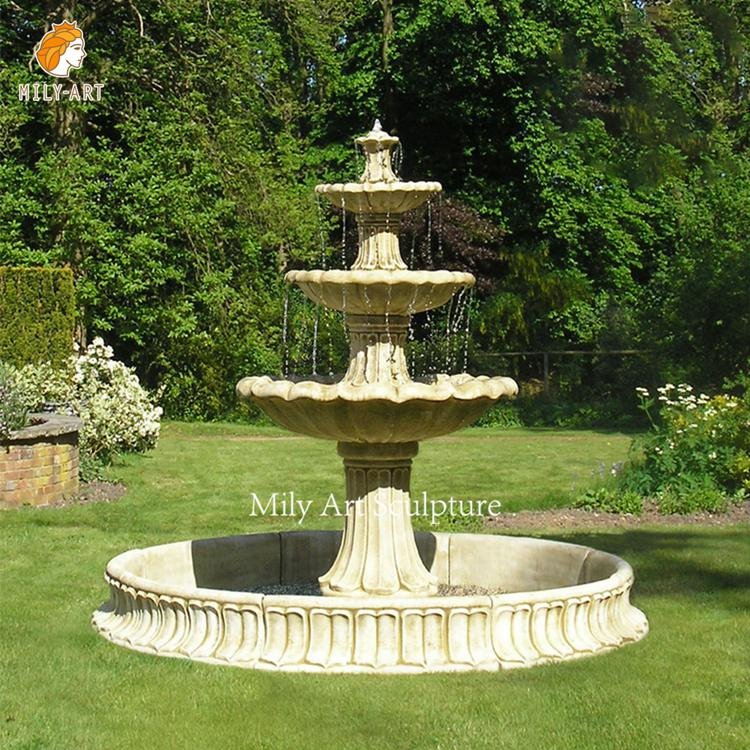The image depicts a weathered, multi-tiered stone fountain in a lush garden. Water pours down in straight lines from four distinct tiers, collecting in a pool at the base. The fountain's aged appearance suggests it has been a centerpiece for quite some time. It sits on a bed of grass, surrounded by various plants, including bushes with white flowers and rose bushes. In the background, large, dense trees cover much of the sky, with an old brick planter housing some of the shrubbery. There’s also a hidden fence and a visible path weaving through the garden.

Notably, in the top left corner of the image, there's a logo featuring a crowned figure and the text “Millie Art.” The words “Millie Art Sculpture” are inscribed at the base of the fountain, attributing the creation to Millie Art. The color of the fountain is predominantly gray with subtle white and yellow hues, blending harmoniously with the vibrant greenery of the yard.